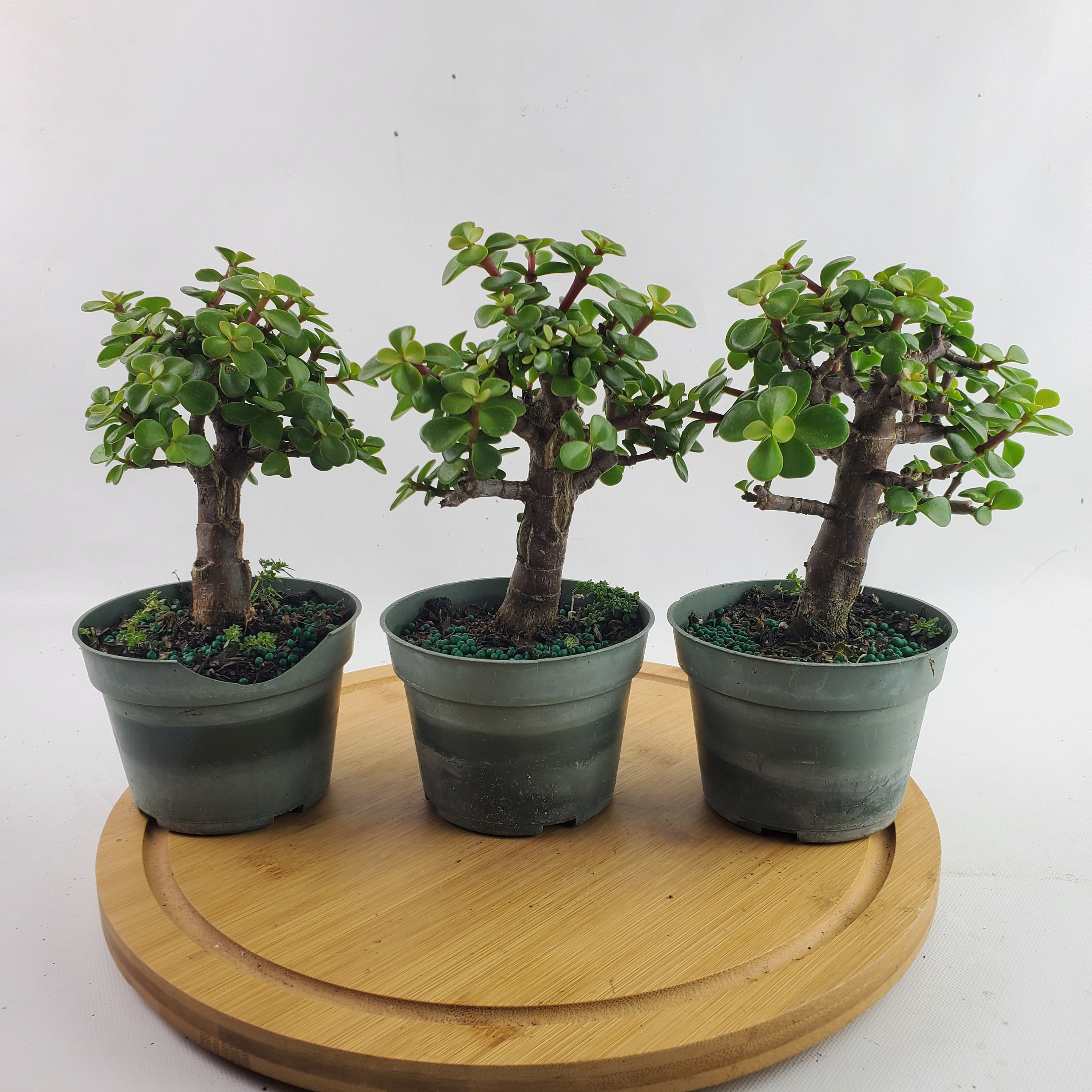The image features three small, bonsai-like trees, each housed in a dark grayish-green planting pot. These pots are lined up side by side on a medium-light wooden circular platform, which has a groove around its edge, resembling a cutting board designed to capture liquids. The pot on the left has a noticeable chip missing from its top lip, while the other two pots are intact but show signs of being dirty. The trees themselves, which have thicker trunks and stalks, sport a lush array of green leaves that range from light to dark shades, giving them a succulent-like appearance. The scene is set against a simple, off-white studio background, enhancing the focus on the trees and their containers.